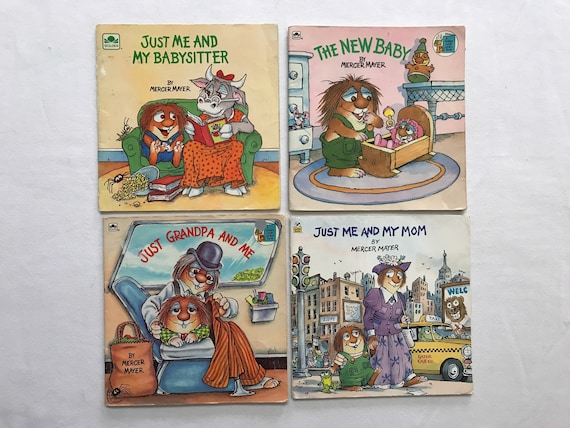This image features a quartet of Little Critter books by Mercer Mayer, arranged in a square against a light gray background. The book in the upper left corner is "Just Me and My Babysitter," which depicts Little Critter sitting on a sofa with his cow babysitter, reading a book together. In the upper right corner is "The New Baby," showing Little Critter standing over a cradle, gazing at his baby sister. The bottom left book is "Just Grandpa and Me," illustrating Little Critter and his grandfather riding a bus with Little Critter facing the viewer. Lastly, the bottom right book is "Just Me and My Mom," where Little Critter is walking hand-in-hand with his mom along a sidewalk. Each cover features Little Critter, an indeterminate rodent-like animal, interacting with family members in various everyday scenarios.